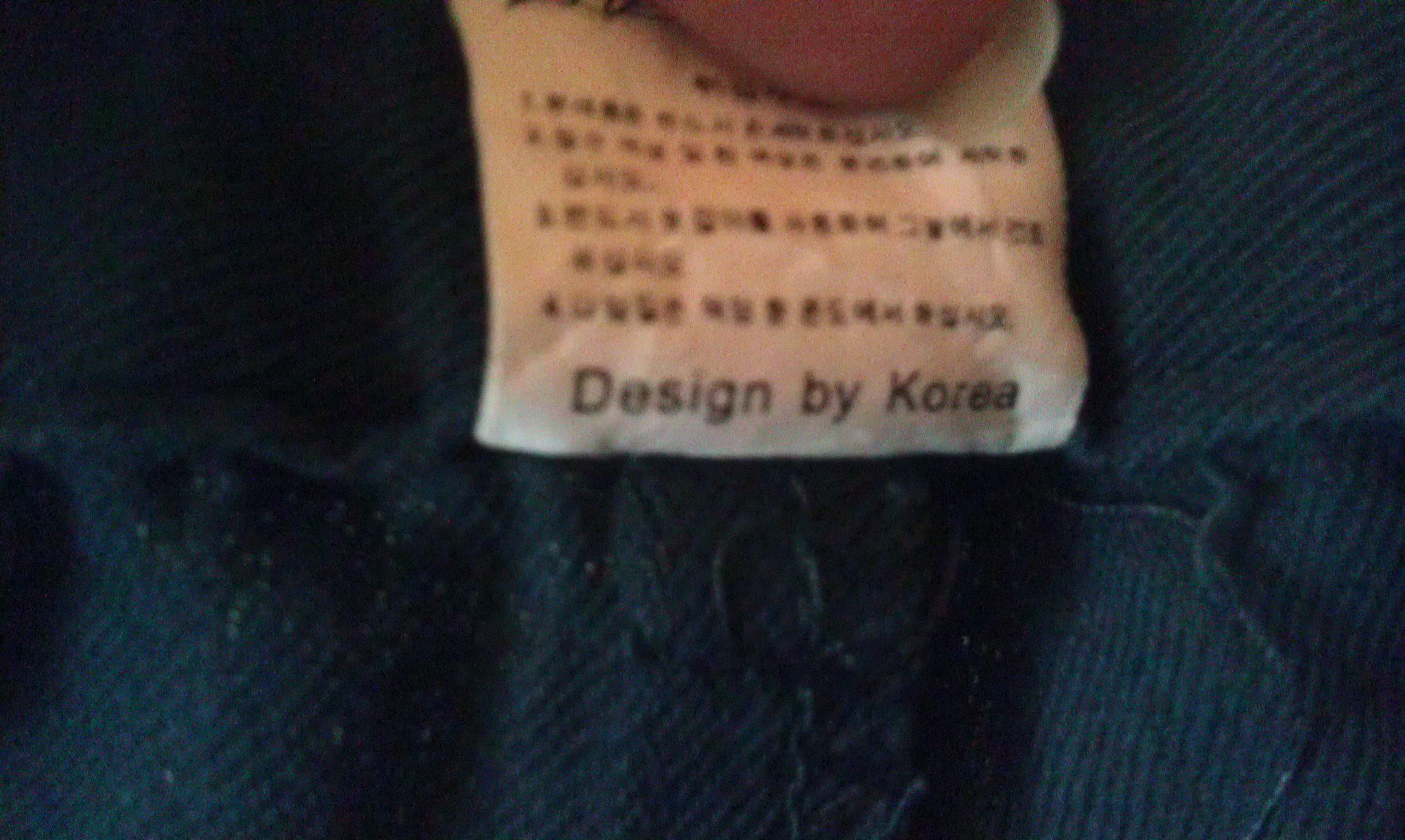This image features a close-up view of a well-worn piece of green, textured fabric with visible pilling and loose threads. A thumb is pulling up a white, square tag that displays both English and Korean text, with "Design by Korea" written in black letters. The tag itself appears aged, displaying waviness and dents. The fabric appears thick, possibly woolen or cotton, with ribbed lines enhancing its texture. Despite the close-up perspective preventing identification of the exact garment type, the detailed focus reveals the worn and textured state of both the material and the tag.